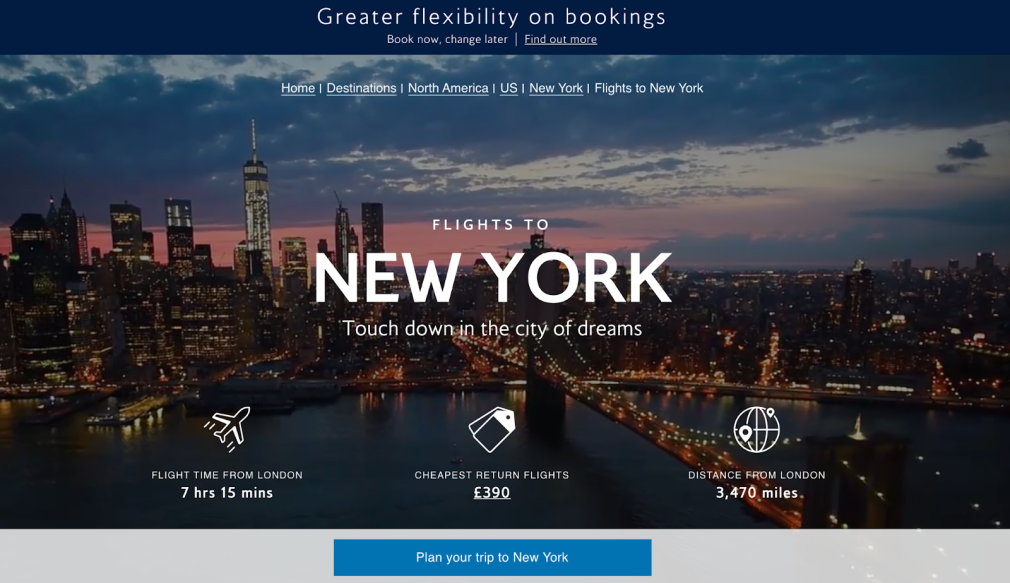Here's a detailed and cleaned-up caption for the given image description:

---
At the top of the web page, there is a dark bluish horizontal bar displaying the phrase "Greater flexibility on booking" in prominent font. Beneath this, in smaller font, is the text "Book now, change later," accompanied by an underlined "Find out more" link, separated by a vertical line.

Below the bar, the main content features a captivating image of a city skyline viewed from the water. An illuminated bridge extends into the city, with a prominent taller building showcasing a brightly lit tower surrounded by several other buildings.

Above the image, a navigation menu includes links such as "Home," "Destinations," "North America," "U.S.," "New York," and "Flights to New York," with "Flights to New York" highlighted but not underlined. Immediately below this menu is the tagline "Touchdown in the City of Dreams."

Further down, an icon of a plane is displayed along with information that the flight time from London to New York is 7 hours and 15 minutes, abbreviated as "7hr 15min." To the right, the page shows the cheapest return flights listed at £390 and the distance from London to New York is noted as 3,470 miles.

At the bottom of the section, there is a grayish bar featuring a medium blue button with white lettering that reads "Plan your trip to New York."
---